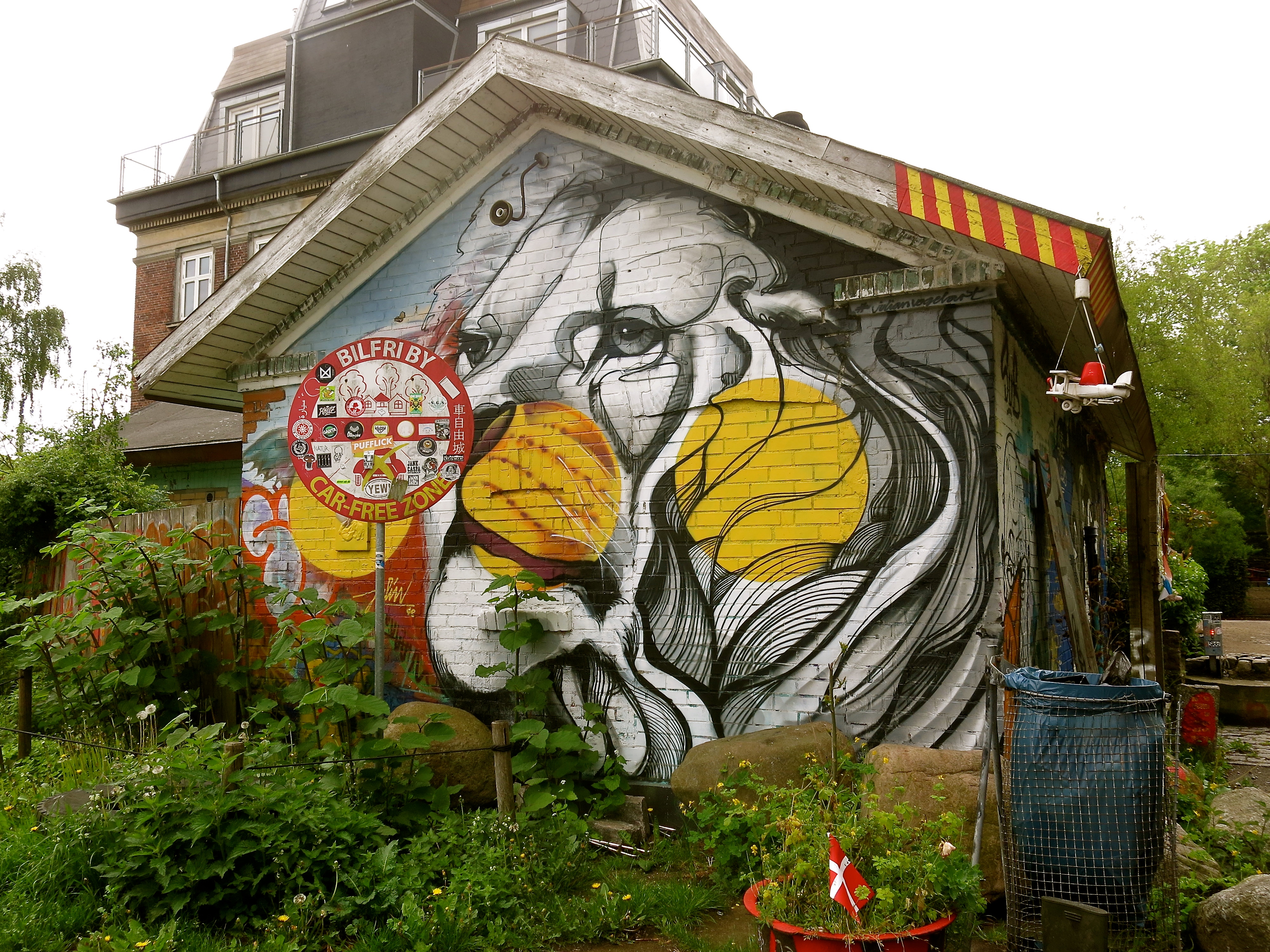This photograph showcases a unique and artistically adorned house. The entire front side of the house is dominated by a striking mural of a lion. The lion's face is primarily rendered in black and white, with selective areas highlighted in the true earthy colors of a lion, featuring tan brown fur and a dark nose. The mural spans the entire wall, creating an eye-catching focal point for the structure.

In the foreground, there is a lush garden filled with various plants and small blooming flowers, adding a touch of nature and color to the scene. A pole with a round sign emerges from the greenery, though the sign is partially obscured by a collection of stickers. The visible text reads "bill free by," followed by what appears to be "car free zone."

Overlooking this picturesque scene is a larger, nondescript structure set against a backdrop of a gray, overcast sky, providing a contrasting background to the vibrant and detailed artwork of the lion.